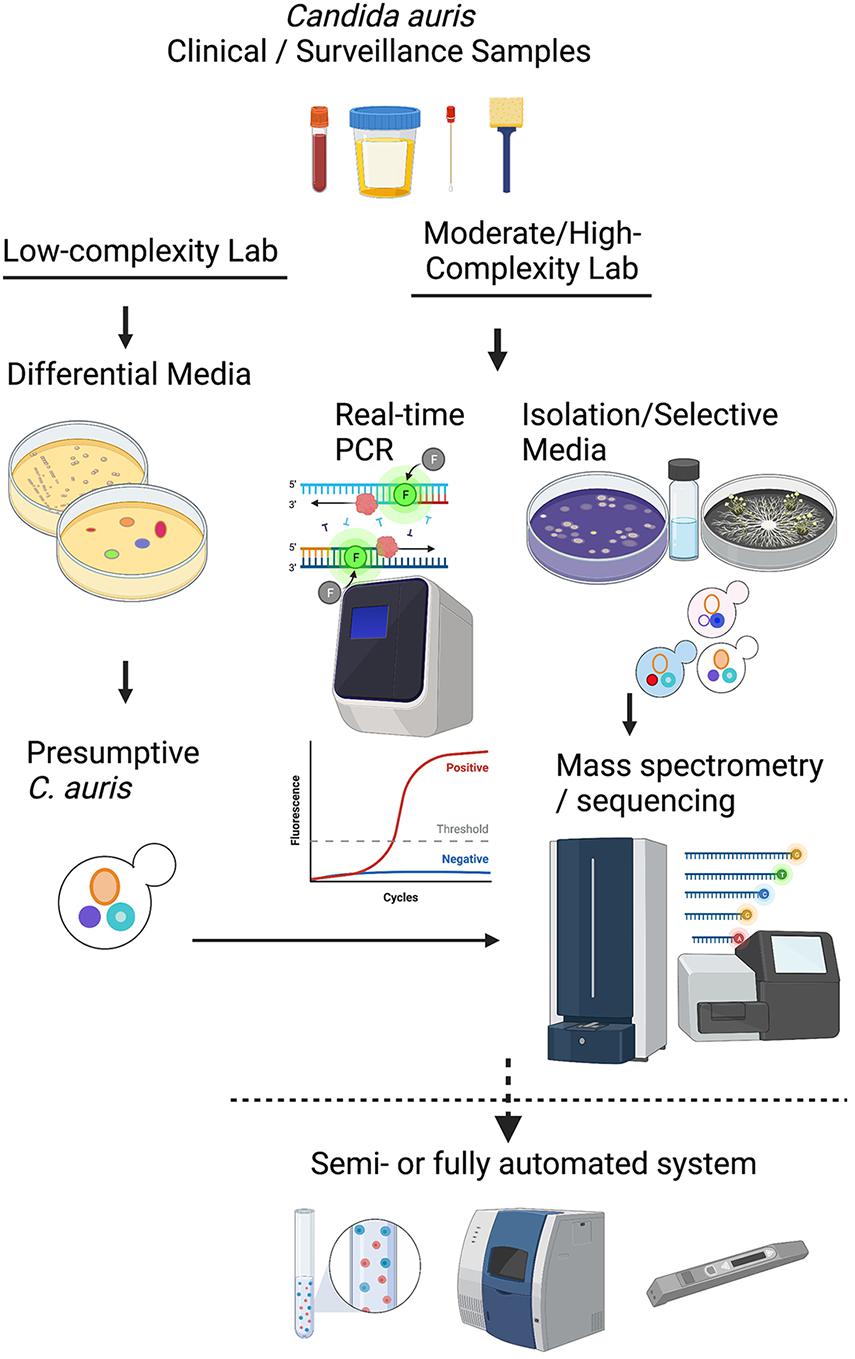This vertical flowchart, headed by the bold and italicized title "Candida auris," intricately details the workflow for processing clinical/surveillance samples using lab equipment. Below the title, clinical/surveillance sample images include a red test tube, a bucket with yellow liquid and blue top, a pipette, and a brush, illustrating the beginning steps. 

Two arrows guide the process into two distinct lab complexity paths: a low-complexity lab and a moderate/high-complexity lab. On the left side, for low-complexity labs, the flowchart leads to differential media, visually represented by Petri dishes with colorful, rainbow-like dots and plain white dots, subsequently pointing towards a presumptive C. auris result. This pathway eventually converges with the high-complexity lab side after additional steps.

On the right, the moderate/high-complexity lab path first indicates real-time PCR, shown with computer-analyzed cell images. Following this, it branches into isolation/selective media, depicted by a test tube and Petri dishes in purple and black featuring visible colonies. The next step on this path is mass spectrometry/sequencing, symbolized by detailed computational analysis on a computer screen.

Both paths ultimately funnel into a semi or fully automated system, marked by a dashed line below the mass spectrometry/sequencing section, providing a comprehensive and detailed visual guide on lab procedures for identifying Candida auris.